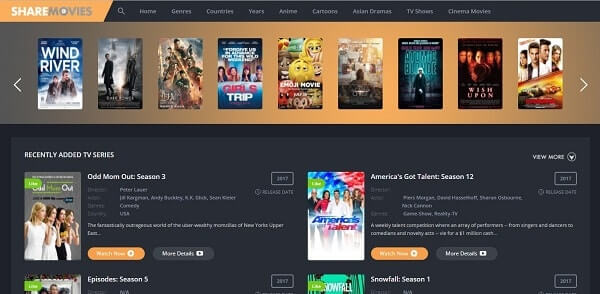The image features a user interface layout with distinctive sections. At the top left, there is an orange box with a diagonal right side that displays the text "Sherry and White and Movies and Dark Grave." Adjacent to it, on the right, is a vertical black bar featuring a menu with a magnifying glass icon followed by options labeled "Homes," "Genres," "Countries," "Years," "Anime," "Cartoons," "Asian Drama," "TV Shows," and "Cinema Movies."

Beneath this menu are several different movie titles arranged in a horizontal scroll. From left to right, the titles include "Wind River," followed by two titles that are too blurry to discern, "Girl Trip," "The Emoji Movie," another blurry title, "Atomic Blonde," "Wish Upon," and the last one which is also too blurry to identify. Flanking these titles are navigation arrows pointing left and right, allowing for scrolling through the movie selections.

Below this section is a gray box that highlights recently added TV series, with specific reference to "Odd Mom Out Season 3" in the top left corner.